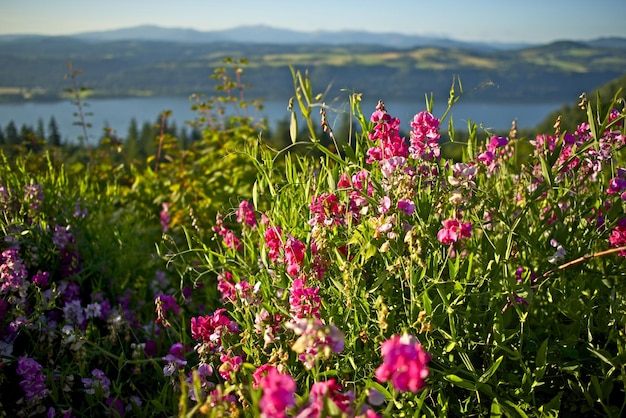The image captures a vibrant outdoor scene featuring a lush expanse of wildflowers and greenery. The foreground is dominated by a striking patch of pinkish-fuchsia flowers, contrasted by clusters of purple blooms on the left. The flowers and surrounding plants are bathed in sunlight, highlighting the vividness of the scene. In the background, you can discern a body of water, possibly a lake or river, with its far shore revealing hilly terrain that leads up to a range of mountains. These mountains appear dark at their base but shift to a bluish hue near the peaks. The sky above is hazy and overcast, exhibiting a gradient of light to darker blue from left to right. The overall feel of the image suggests a sunny day in late spring or early summer, with everything looking exceptionally green and lively.